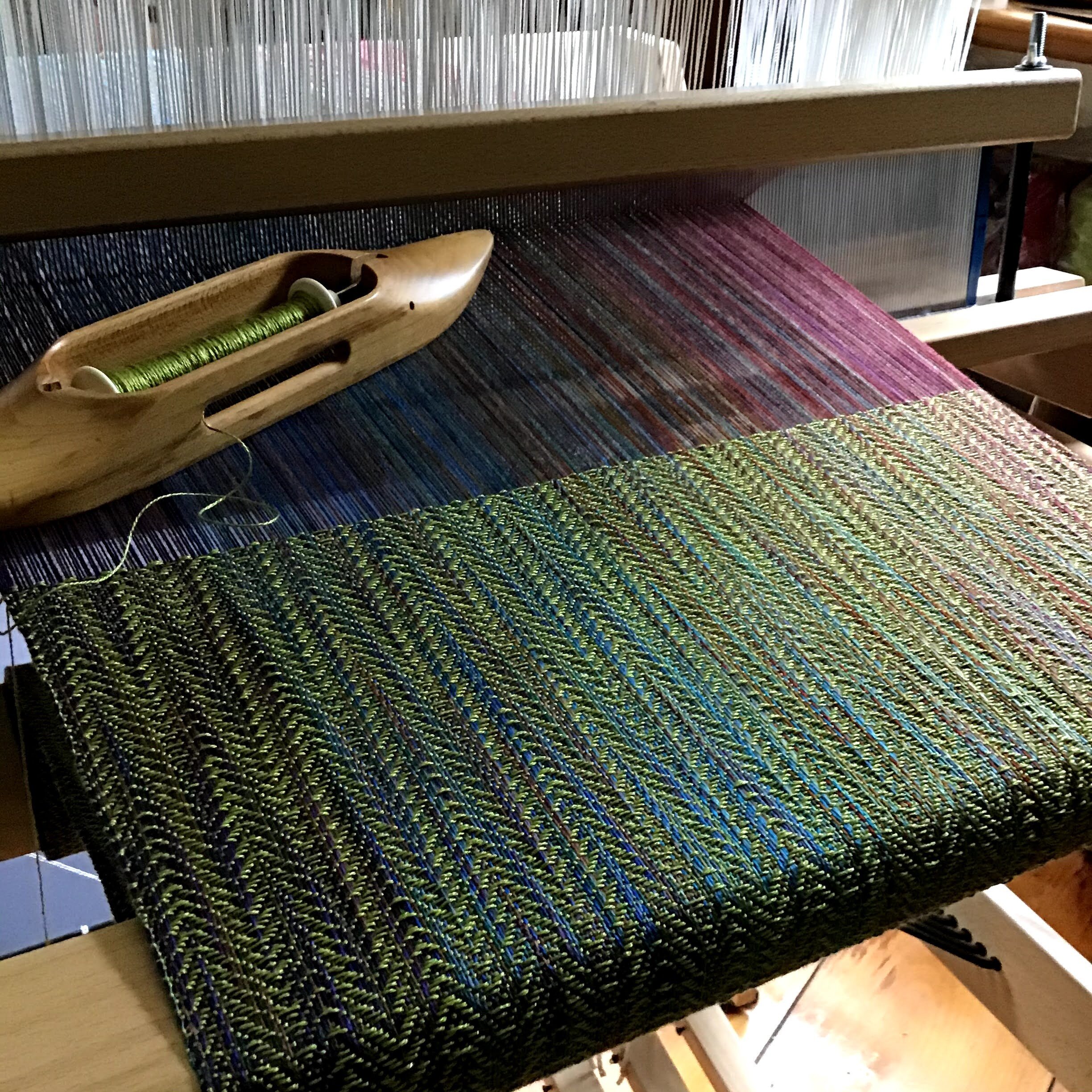This detailed color photograph depicts an indoor view, looking down at a weaving loom in progress, set against a wooden floor. The loom's light-colored frame contrasts with its intricate weaving, with vertical dark purple threads strung along its structure. In the loom's bottom section, a herringbone pattern of dark green and blue fabric is emerging, woven against red threads, and partially completed about halfway up. A wooden shuttle, resembling the shape of a shoe with an open oval center, rests on the top left of the loom, containing a spool of green thread. This thread cascades towards the active weaving area below. Behind the woven area are vertical white strings, and a horizontal wooden pole likely aids the weaving process, contributing to the complex and beautiful fabric being produced. The overall composition underscores the realism and detailed craftsmanship of fabric creation.